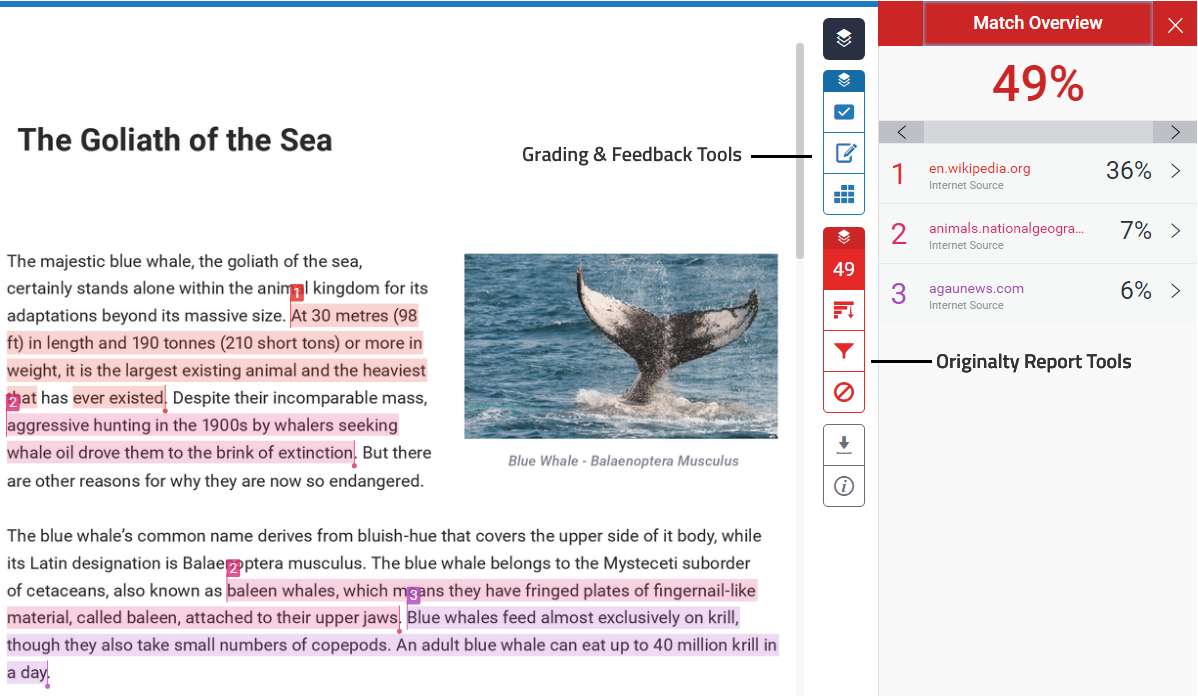**Caption: Blue Whale - The Goliath of the Sea**

On the left side of the image, bold black text reads "The Goliath of the Sea," accompanied by highlighted text elements. Below this title, the description elaborates: "The majestic blue whale, the Goliath of the Sea, certainly stands alone within the animal kingdom for its adaptation beyond its massive size. At 30 meters (98 feet) in length and 190 tons (210 short tons) or more in weight, it is the largest existing animal and the heaviest that has ever existed." This segment is highlighted in a light red color labeled as number 1.

The next section, highlighted in light pink and labeled as number 2, addresses the challenges faced by blue whales: "Despite their immense size, aggressive hunting in the 1900s by whale-seeking whalers drove them to the brink of extinction. But there are other reasons why they are now so endangered." Further details include the origin of the blue whale's name, derived from its bluish hue and Latin designation, Balaenoptera musculus. Blue whales belong to the Mysticeti suborder of cetaceans, also known as baleen whales, characterized by fringed plates of fingernail-like material called baleen attached to their upper jaws.

Another section highlighted in light purple and labeled as number 3 discusses the blue whale's diet: "Blue whales feed most exclusively on krill, but they also consume small numbers of copepods. Adult blue whales can eat up to 40 million krill a day."

On the right side of the image, at the top, it states "Match Overview" with a 49% metric in red. Below this, sources are listed: "1. Wikipedia – 36%, 2. Animals.NationalGeographic – 7%, 3. Aqua News – 6%." At the bottom, tool options are displayed: "Filter," "Originality Report Tools," "Grading and Feedback Tools."